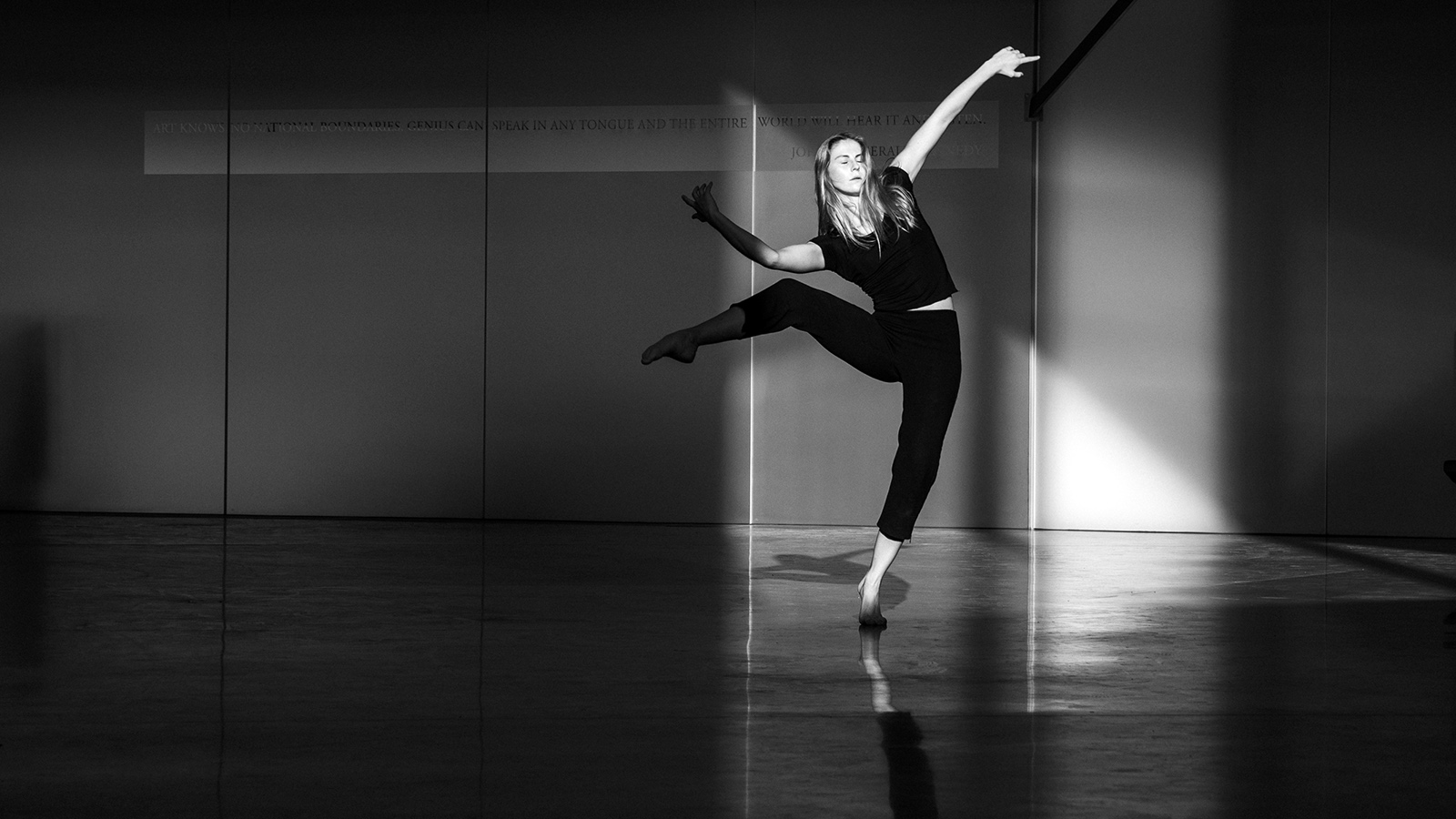In the grayscale image, a female dancer is captured mid-movement in a spacious, empty room marked by minimalist design. She is barefoot, adorned in an all-black outfit consisting of a short-sleeved top and calf-length pants or leggings. Her long, loose hair flows around her as she balances on one leg with her other leg cocked to the side, striking a pose that blends elements of ballet and interpretive dance. Her hands are extended to the sides, and her eyes are closed, suggesting deep concentration.

The room itself is bathed in varying shades of gray, with little bits of white and lighter gray adding subtle contrast to the bare walls. The highly reflective floor catches and mirrors the dancer’s silhouette and her shadow looms behind her. Along the top of the walls, partially obscured text or a quote can be seen, saying "speak innately tongue and their entire world will hear it," though some parts remain unreadable due to reflections. A single ray of light pierces the monochromatic scene, illuminating the dancer while leaving the rest of the room in shadow. This striking light source appears to come from a window, placing the dancer as the focal point of the evocative scene.